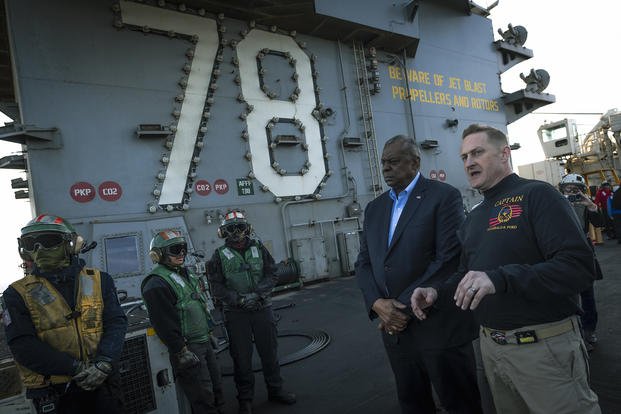The image depicts a scene aboard an aircraft carrier, likely focusing on its Conning Tower, identified by a large white number "78" prominently displayed. The background is characterized by an assortment of industrial equipment and electrical machinery fastened to the gray steel structure of the tower. Additionally, a warning in yellow text reads, "Beware of Jet Blast Propellers and Rotors," and satellites can be seen in the upper right-hand corner.

In the foreground, five individuals are present. Three military personnel stand to the left, donned in protective gear including black goggles, helmets in red and gray, face coverings, and colored vests in shades of green and yellow, along with dark pants and black sleeves. Adjacent to them is an African American man, possibly the Secretary of Defense, wearing a black jacket over a blue open-collar shirt, his hands crossed in front of him. To his right, an older white man—potentially the Captain or air boss—is seen wearing a dark sweater with the word "Captain" in gold above an American flag emblem on his left chest, complemented by tan pants. He appears to be conversing with the Secretary of Defense, adding an air of seriousness to the scene.